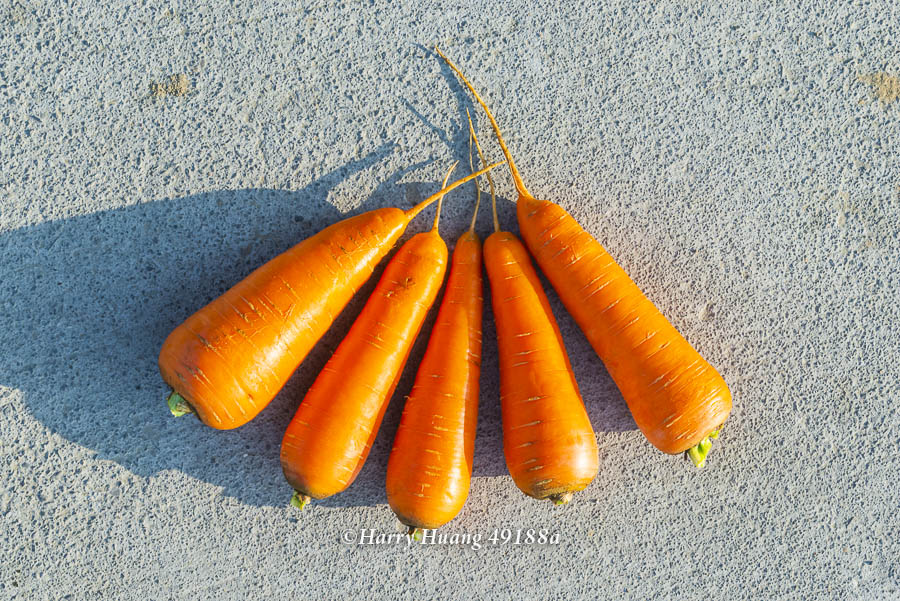The image features five vibrant, full carrots arranged in a fan-like pattern on a light gray, mottled concrete surface. The carrots, varying in width, showcase a thick and sturdy one on the far left, three moderately sized ones in the middle—with the center carrot being slightly thinner at the bottom—and a moderately thick but taller carrot on the far right. They have been freshly trimmed, leaving only small green stems protruding. Tiny rootlets are visible at the ends of each carrot. The lighting comes from the right, casting shadows to the left. Below the carrots, in white text, it reads: "© Harry Hwang 49188a."